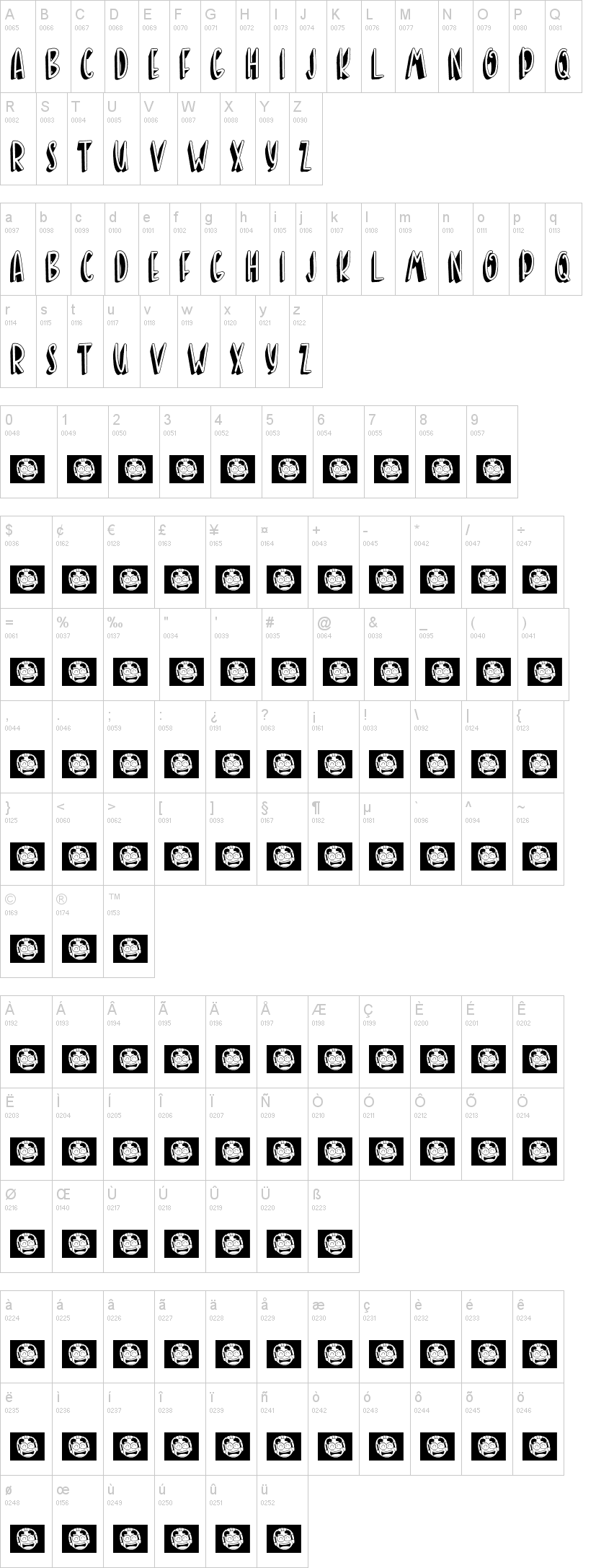The image depicts a highly detailed, monochromatic page divided into several distinct sections. At the very top, the entire alphabet is displayed in a unique, cartoon-style font. Each letter, from A through Z, is presented on a light gray rectangular tab. The tabs bear numbers written in a standard, typical font, while the letters themselves are rendered in a stylized, comic book-like appearance.

Below the alphabet section, the page features multiple boxes, each containing an illustration of a cartoon person with a visibly stressed expression. These boxes seem to offer various numerical options at the top. Beneath the numbers, a variety of symbols are shown, including currency symbols, punctuation marks, and additional letters. The layout and diversity of the typesetting suggest a dynamic range of typographical elements designed to add flair and emphasis to written content.